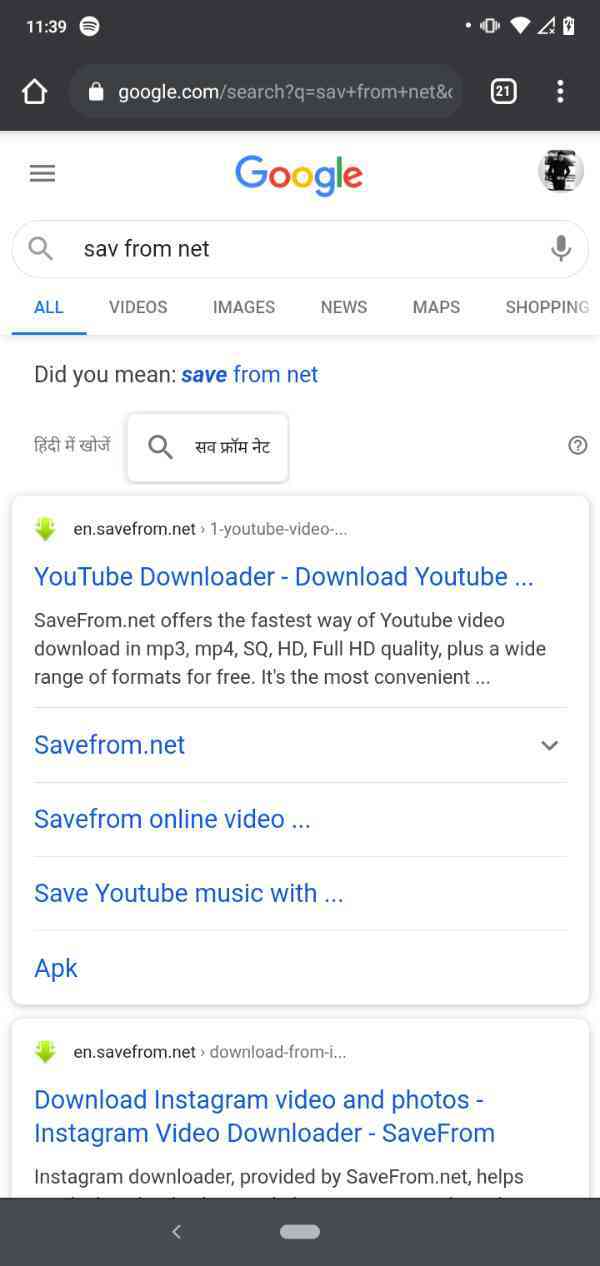A detailed descriptive caption for the image could be:

"Captured from a cell phone screen, this image displays a Google search page where the user has entered 'SAV from net.' As the search term is incomplete, Google suggests 'SAVE from net,' highlighted in blue as a clickable correction. Below the search bar, text appears in what seems to be Korean or another Asian language, implying the search might also be related to international content. Scrolling down slightly, a prominent result appears for "en.savefrom.net," labeled as a YouTube downloader. It promotes SaveFrom.net as the fastest method to download YouTube videos in various formats such as MP3, MP4, SQ, HD, and full HD, emphasizing its convenience and wide range of available formats. Item descriptions continue with the inclusion of 'Save from online videos,' 'Save YouTube music,' and 'APK,' indicating additional functionalities related to video and music downloading."